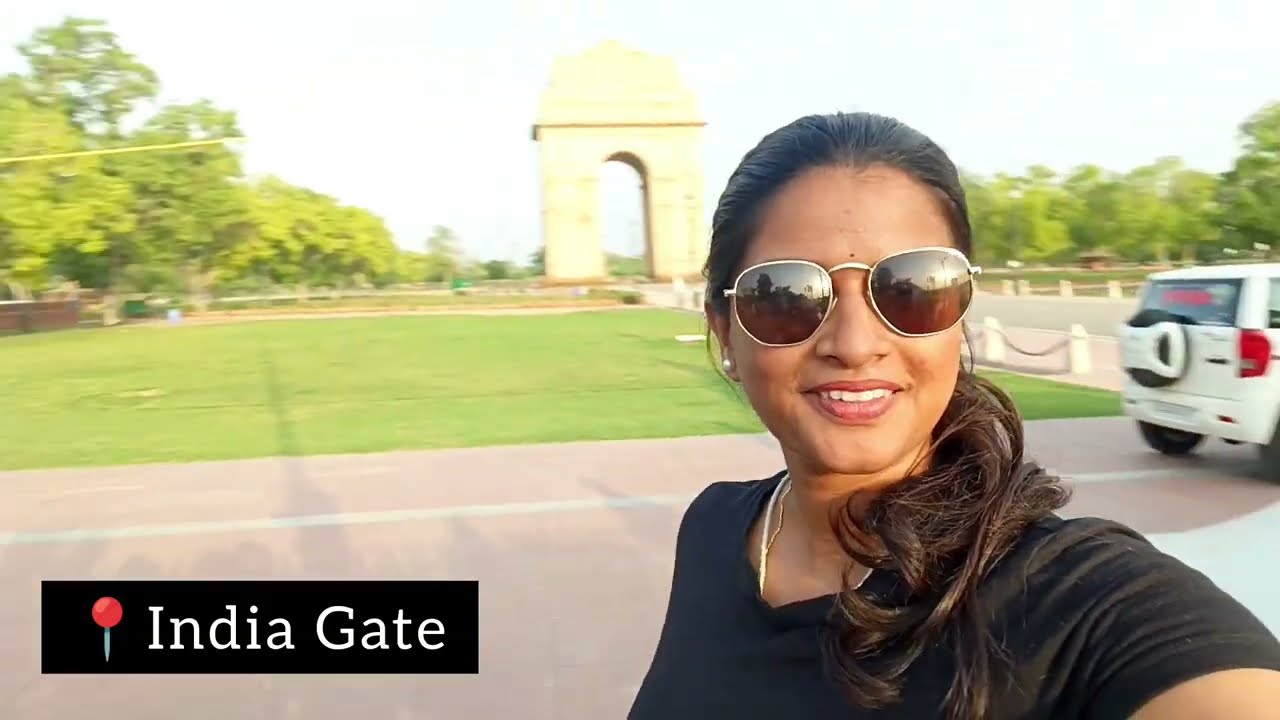In a brightly lit daytime selfie, a woman with long, black hair tied back in a ponytail that curls at the ends and falls over her right shoulder poses in front of the iconic India Gate. She’s dressed in a black shirt, wearing large, dark sunglasses, and sporting red lipstick while smiling. The backdrop features a significant yellow arch, recognized as India Gate, along with a mix of white bollards linked by chains lining a path, possibly a pedestrian walkway. Behind her, there is a distinct white SUV, identified as a Suzuki, parked nearby. Additionally, green leafy trees and a paved road can be seen, with a lit, light blue sky above. At the bottom left corner of the image, a marker pin with the label "India Gate" is visible, encapsulated in a black rectangle.